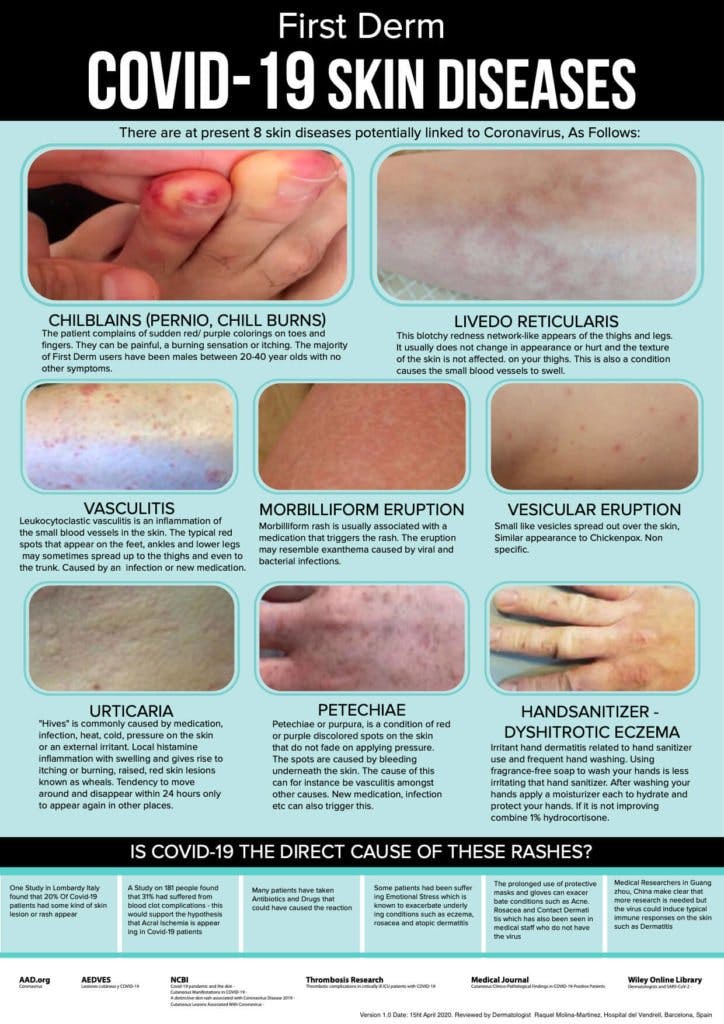The image is an educational pamphlet titled "First Derm COVID-19 Skin Diseases," prominently displayed in white text on a black background at the top. The rest of the pamphlet has a light blue background. The central content consists of eight photographs, each depicting a specific skin condition potentially linked to COVID-19. The conditions include chilblains (pernio or chill burns) on toes and fingers, livedo reticularis, vasculitis, morbilliform eruption, vesicular eruption, urticaria, petechiae, and hand sanitizer-induced eczema. Each photograph is accompanied by descriptive text, some of which appear to be in Spanish. At the bottom of the pamphlet, there is a poignant question in white font: "Is COVID-19 the direct cause of these rashes?" This section also contains further discussion and encourages readers to consult a healthcare professional if they experience any of these symptoms.